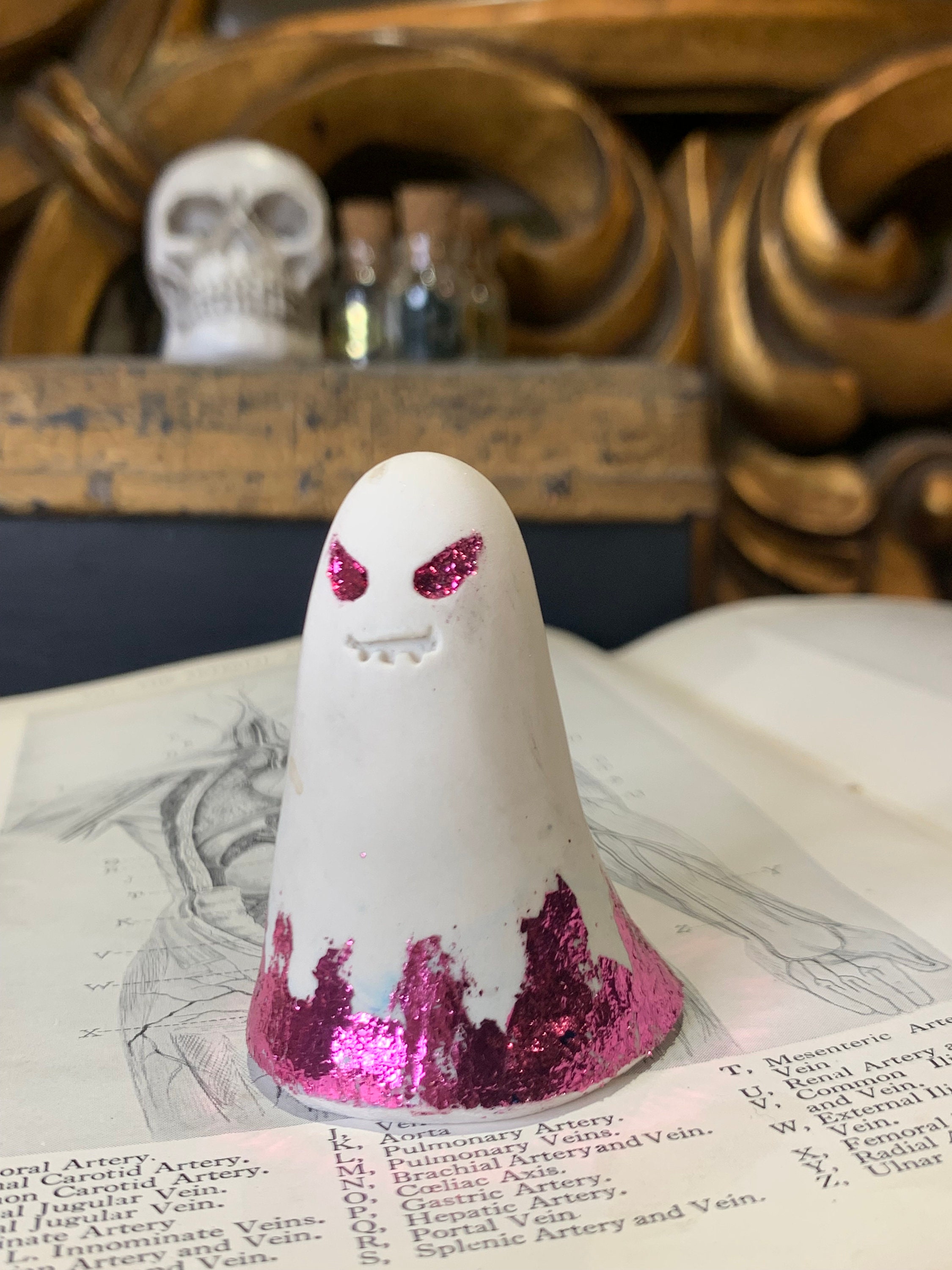The image features a detailed and eerie Halloween setup. In the background, a white skull with a closed mouth and intact teeth is prominently displayed beside three short glass bottles sealed with corks. These bottles and the skull rest on a wooden table. Behind them, a large, ornate gold piece with intricate carvings adds depth and richness to the scene. In the foreground, a handmade ghost decoration steals the spotlight. This ghost, crafted to resemble a spectral figure, is entirely white with slanted, pink glittery eyes giving it an intriguingly sinister but slightly cheerful appearance. Its base is accented with smudged pink glitter, creating a whimsical yet spooky aura. The ghost sits atop a book featuring human anatomy illustrations, suggesting a playful contrast between science and the supernatural. The overall effect is one of a meticulously arranged, atmospheric Halloween display that blends elements of study and festivity.